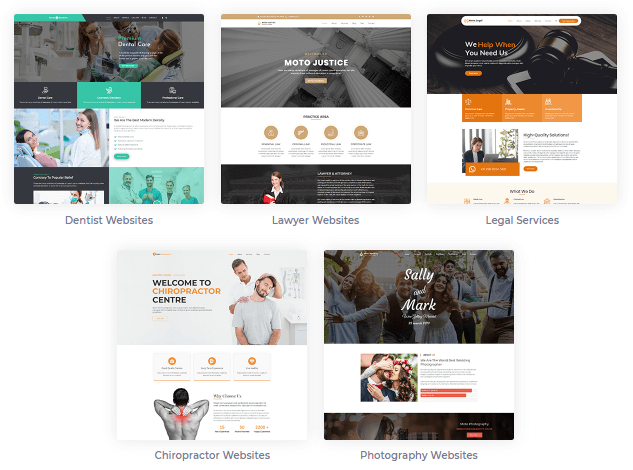The image depicts a webpage dedicated to referral services, organized into two horizontal rows. The design has a clean, white background that enhances readability. 

In the first row, there are three sections, each with a header and an illustrative image directly above the text:
1. **Dentist Websites** - Displayed in bold black text, this section features an image showcasing various dental websites. 
2. **Lawyer Websites** - Similarly, bold black text introduces this section, paired with a relevant image that provides links to different lawyer websites.
3. **Legal Services** - The section header in black text is supplemented with an image that offers insights into various legal services.

In the second row, there are two sections:
1. **Chiropractic Websites** - The header "Chiropractic Websites" introduces the content, and underneath, the text "Welcome to Chiropractor Center" gives a brief overview of chiropractic services. This section is illustrated with a relevant image.
2. **Photography Websites** - The final section, headlined "Photography Websites," includes the names "Sally and Mark" and displays examples of their photography work.

Each section is carefully categorized with a combination of descriptive text and visual aids, ensuring a user-friendly interface for finding specialized referral services.